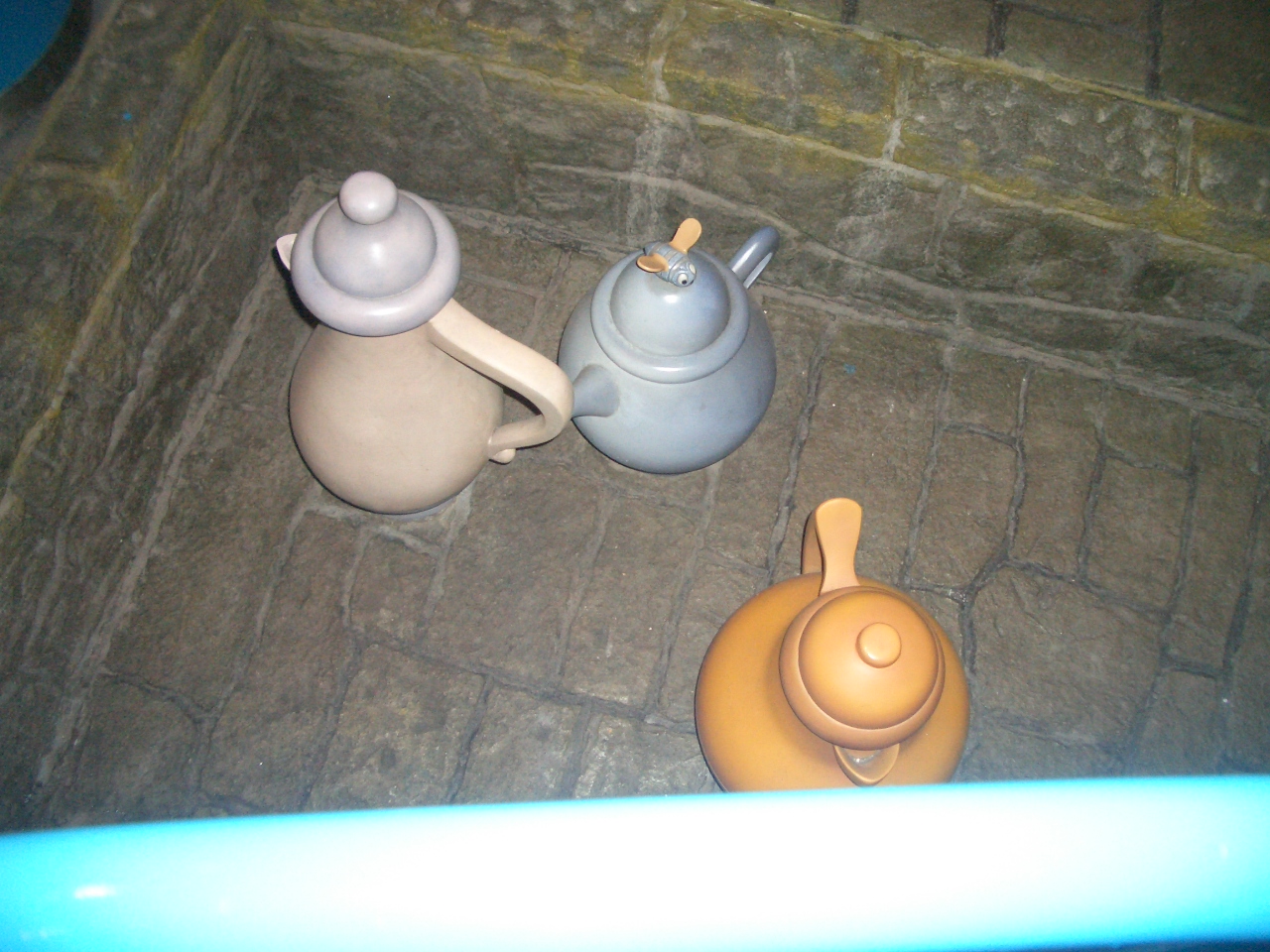The image captures three small ceramic teapots placed within a brick enclosure that has the appearance of a kiln or an aged stone corner with worn, dark brown, misshapen bricks. The bricks are mottled in color with hints of moss, giving the top layer a greenish, worn texture. A disjointed blue line cuts across the bottom 15% of the image, possibly an unintended reflection or flash artifact from the camera.

Starting from the left, the first teapot is a charming mix of pink and purple, with a pinkish handle and body, and a bluish-purple, round lid with a little knob on top for easy lifting. The middle teapot stands out with its squat, round shape and a light blue hue. Atop this teapot sits a tiny ceramic figure resembling a bee, detailed with white and black eyes, and orange-tinted wings. To the far right, a vibrant orange teapot exhibits a classic design with a neatly fitted lid and a pouring spout, positioned close to the bottom edge of the image.

The overall impression suggests that these playful and colorful ceramic pots, potentially toys given their small size, were possibly photographed in an impromptu, childlike manner, perhaps with a kid’s digital camera. The absence of human figures or text in the photograph adds a simple yet intriguing narrative, emphasizing the teapots' whimsical presence within the rustic brick backdrop.